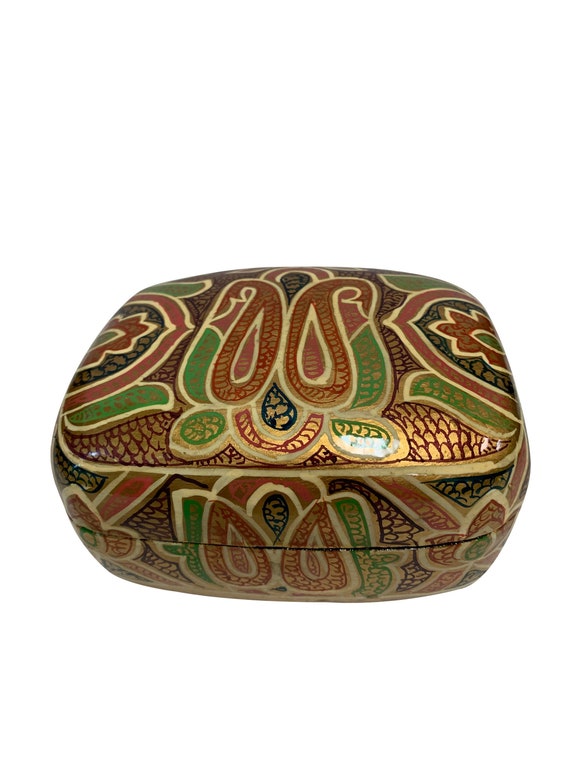The image is a detailed product photo of a small stash box featuring an elaborate and colorful ethnic design. The box, with dimensions appropriate for storing jewelry or knickknacks, boasts a striking red and green color scheme, complemented by accents of gold, black, brown, and tan. The lacquered finish adds a shiny, polished look to the intricate decorations. The box opens up in half, and the lid completely detaches, ensuring easy access to its contents. The top and sides of the box are adorned with swirly patterns and scalloped details, interspersed with vibrant flowers. The front of the box features a central black teardrop shape with intricate squiggles, flanked by similar shapes inverted on either side. Additionally, two prominent round pieces with green leaves hang centrally on the lid, which also displays red flowers with green centers on both sides. The front corners similarly host gold and red flower patterns, creating a cohesive and ornate design that emphasizes both elegance and cultural artistry.